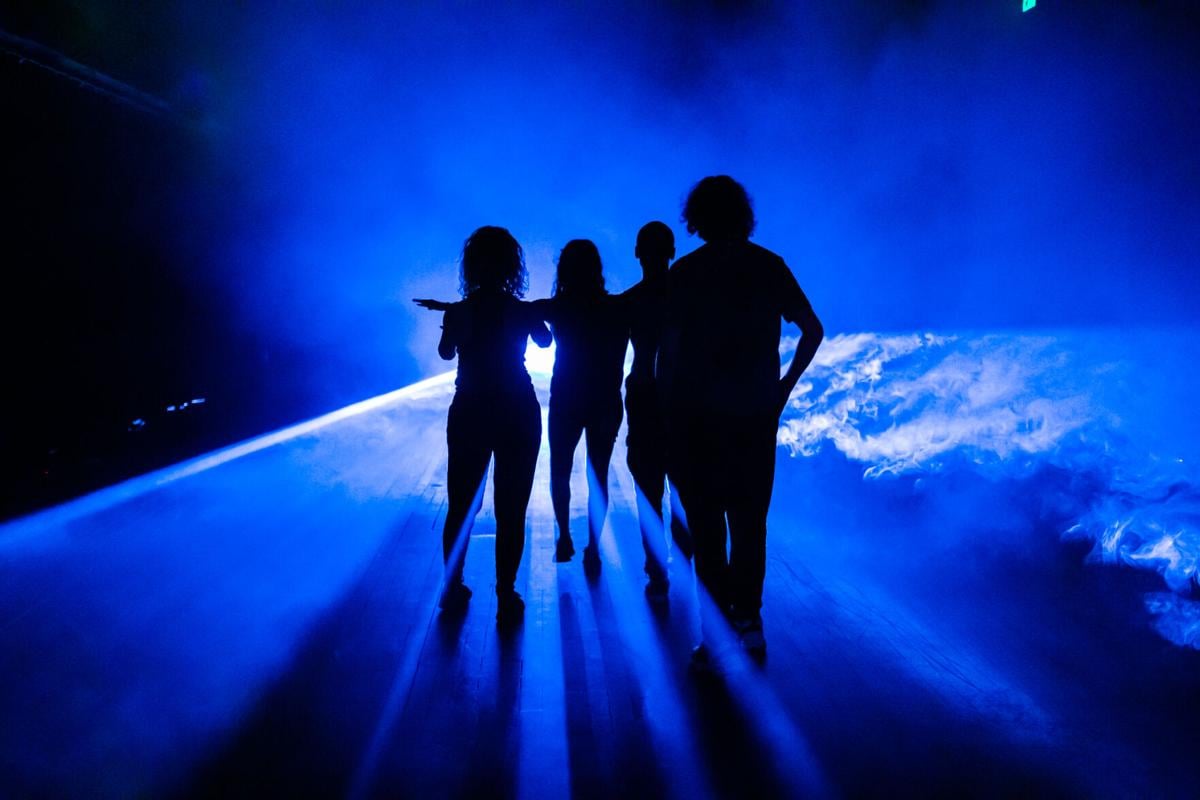This horizontally aligned rectangular image, taken at night, captures a blurry and grainy scene on what appears to be a road or highway. The upper left corner of the image is solid black, transitioning into a blue smoke effect that permeates the rest of the upper portion of the picture. The entire scene has a distinct blue tint, enveloping four silhouetted figures positioned on the road. The silhouettes, suggesting the forms of teenagers, are solid black and seem to be moving away from the viewer toward a bright set of headlights in the distance, facing the light source. The right side of the image hints at snow-covered ground, enhancing the cold, nocturnal atmosphere. The light from the headlights illuminates multiple areas, making the blue smoke or dust around the figures more pronounced, resembling rolling flames or gas. Overall, the image evokes a mysterious and surreal ambiance as the silhouettes walk into the blue-lit night.